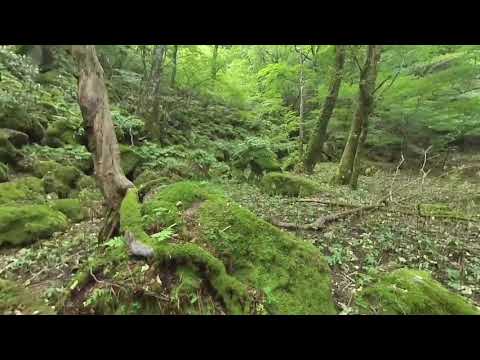This image captures a dense, overgrown forest in the middle of the day, drenched in varying shades of green and brown. At ground level, the scene is dominated by a bare tree leaning to the left, with a conspicuous root emerging from its base. Moss or algae carpets the forest floor, intertwining with the dirt, sticks, and scattered leaves. Clustered around the tree are several hillocks and larger clumps of rocks, all blanketed in lush green moss. The forest itself rises gently on both sides with rocks and vegetation, creating a sloped, textured landscape. In the background, an intricate canopy formed by numerous moss-covered trees provides a vivid backdrop. Patches of sunlight penetrate the dense foliage, adding a touch of brightness. Bushes and small weeds sprinkle the scene, while downed branches lie strewn on the ground, contributing to the natural, untamed beauty of the forest. There is an evident absence of man-made objects and text, leaving the unspoiled essence of nature as the sole focus.